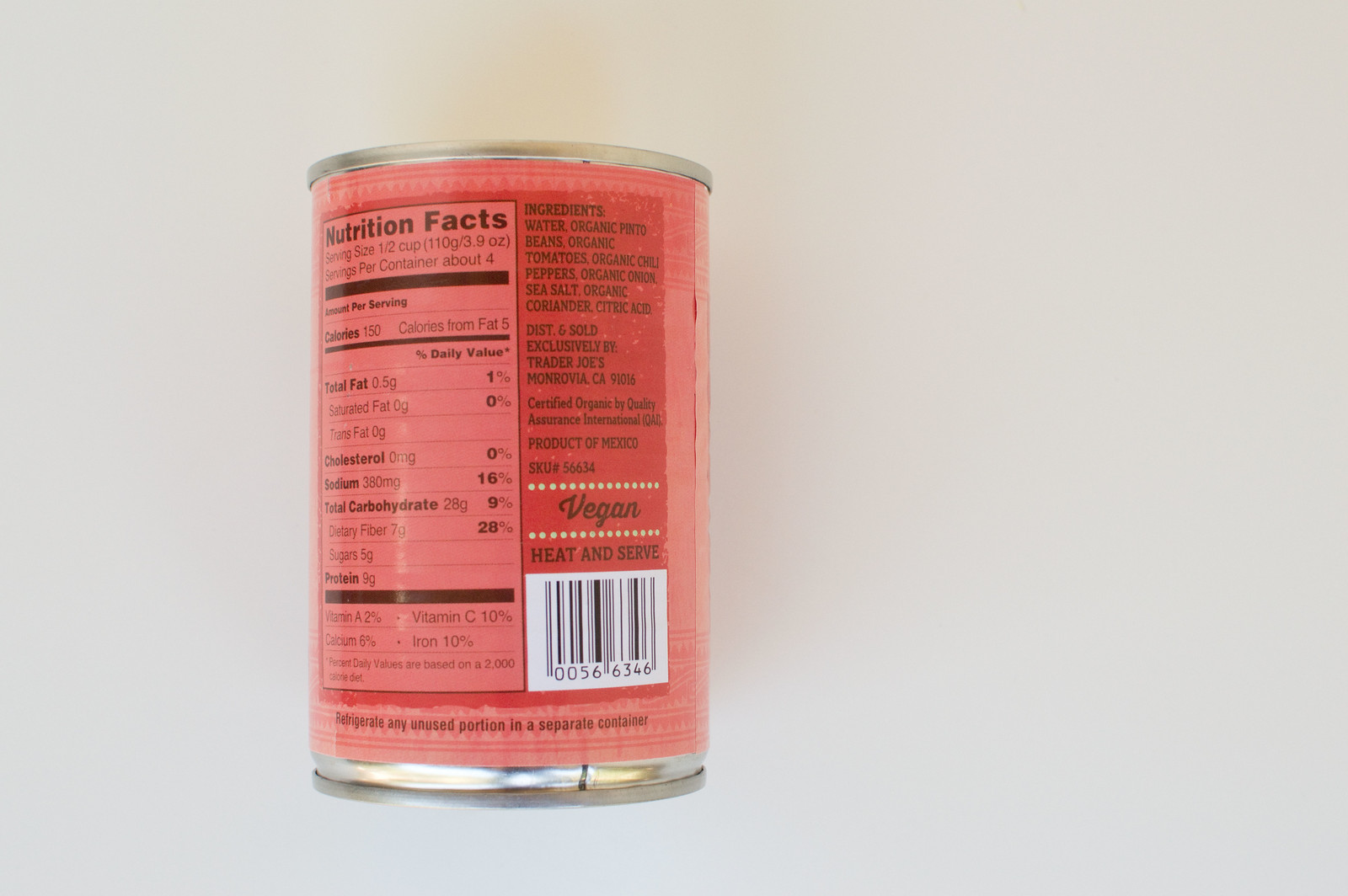This detailed color photograph showcases a single can of food placed on a white surface. The silver can is wrapped in a distinct red and pink label. The can is positioned face down, clearly presenting its label details. On the left side of the label, a comprehensive nutrition facts table lists calories, total fat, saturated fat, trans fat, cholesterol, sodium, total carbohydrates, dietary fiber, sugars, and protein. Additionally, vitamin A, vitamin C, calcium, and iron contents are specified. To the right of the nutritional table, an ingredient list details water, organic pinto beans, organic tomatoes, organic chili peppers, organic onion, sea salt, organic coriander, and citric acid. An unmistakable barcode is also visible. The label further informs that the product is vegan, and suggests it is ready to heat and serve. The can is distributed and sold exclusively by Trader Joe's, headquartered in Monrovia, California.